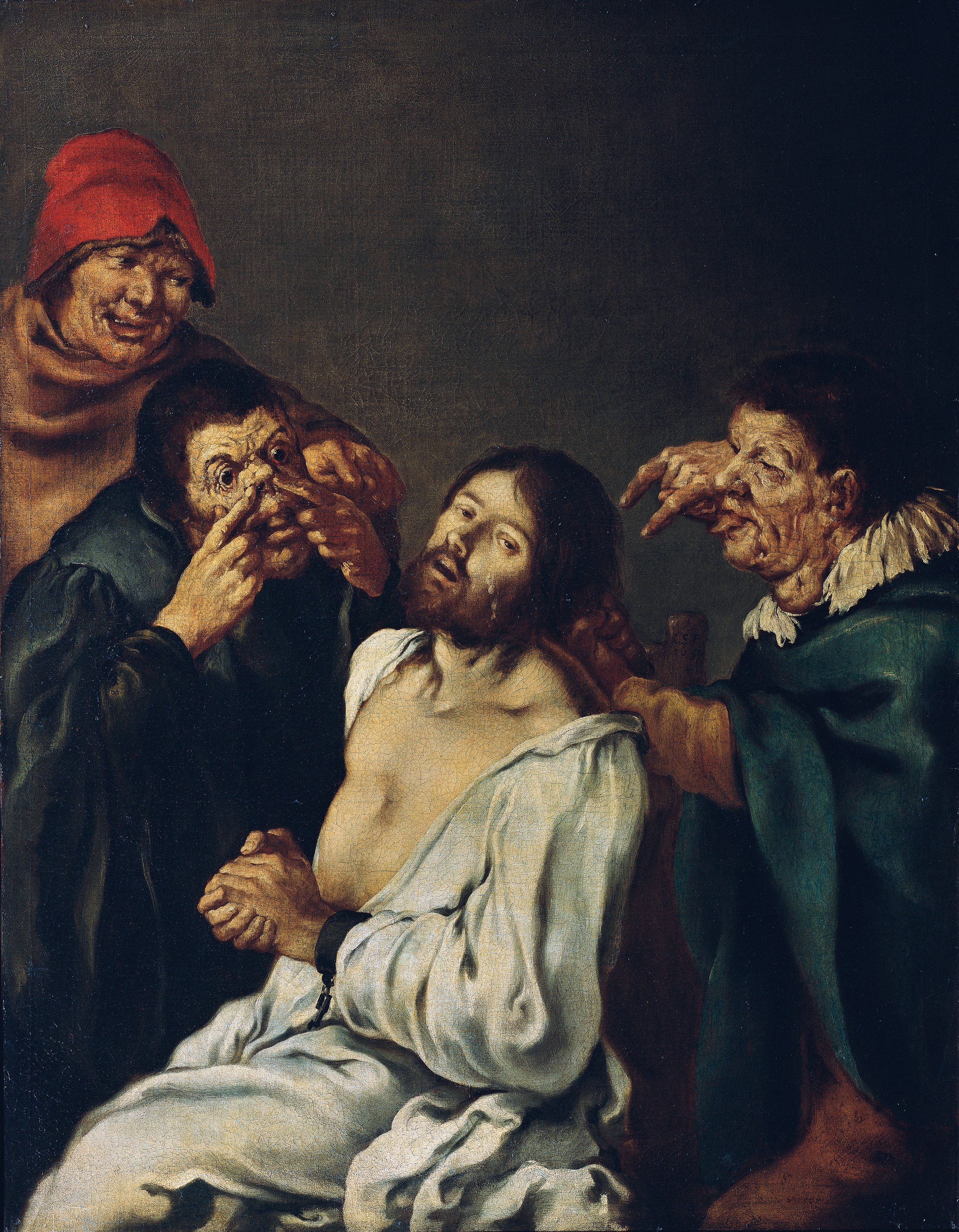This detailed painting, possibly from the Middle Ages or the 1700s, depicts a distressing scene centered around a man in a white, torn robe sitting in a chair. His wrists are bound with shackles, and he clasps his hands in front of his stomach, appearing to be in deep misery and possibly crying. His bearded face, marked with anguish, is turned toward the viewer, as if silently pleading for help.

Surrounding him are three men with grotesque, distorted features that evoke images of lepers. One to his right, dressed in blue, sticks out his tongue while making a vulgar hand gesture with his pinky and index finger extended. Another man to the left, wearing green, makes a pig-nose gesture, pushing his fingers into his nostrils. The final tormentor, behind the seated man and sporting a red hat, looks down at him with a mischievous grin, absorbing the scene with evident enjoyment.

The painting’s background has a brownish-tan hue, enhancing the somber and oppressive atmosphere. The person being taunted and tormented stands out not only because of his central position but also due to his relatively realistic appearance, contrasting with the almost monstrous visages of his tormentors. The primary colors in the scene are white, red, blue, and green, which highlight the figures' clothing and add to the painting's overall impact.